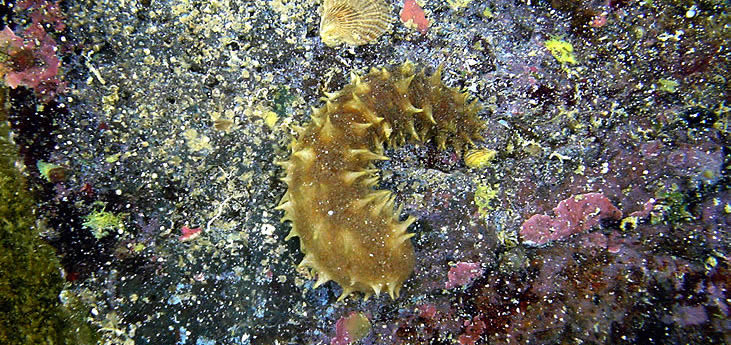The image depicts a spiny, yellowish-brown creature, possibly a worm or sea cucumber, positioned centrally. Its body curves into a 'C' shape and is covered in lighter yellow spikes. Surrounding this creature are numerous cream-colored dots scattered across the surface, which might be sand particles. Above the creature, there is an intact yellow seashell. The background displays various reddish, pinkish, and purplish blotches, resembling coral reef vegetation, adding to the aquatic ambiance. The scene is viewed from above, giving the impression that it is the ocean floor, and the clarity of the water makes it appear almost indistinguishable. The overall palette is dominated by shades of purple, pink, and black, and the image is rectangular.